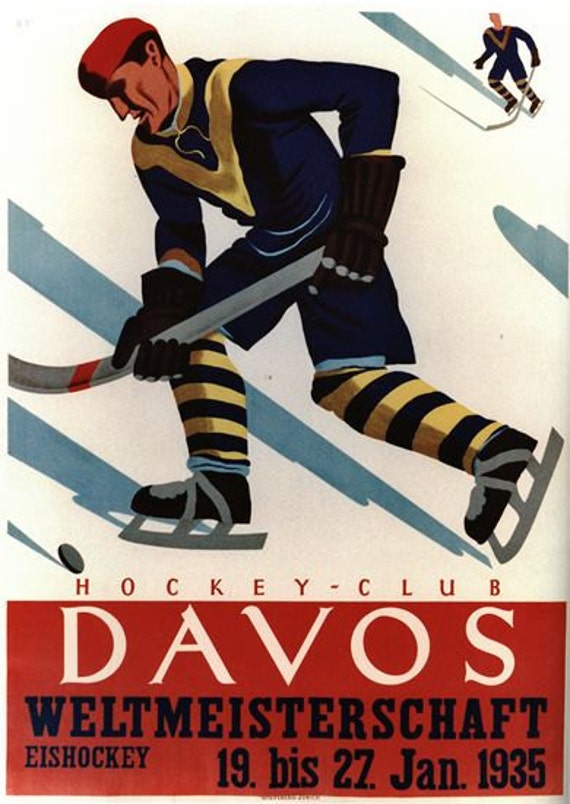This is a highly detailed color poster advertisement for the Hockey Club Davos, promoting the Weltmeisterschaft Ice Hockey tournament scheduled for January 13 to 27, 1935. The central focus of the drawing features a male hockey player in a three-quarter view, predominantly displaying his left side. Dressed in a dark blue uniform with a gold 'V' emblem on the chest, he complements his outfit with blue and gold striped socks and a red cap. The player, who is geared with black gloves and skates, is shown intently looking down at a hockey puck while holding a hockey stick. Shadows add depth to the white background. Additionally, a smaller figure of another hockey player can be seen in the upper right corner. The bottom of the poster presents text in various colors: "Hockey Club" in bold red letters, "Davos" in white letters, and "Weltmeisterschaft, Ice Hockey" in black letters, followed by the event dates “13 BIS 27 JAN 1935.”